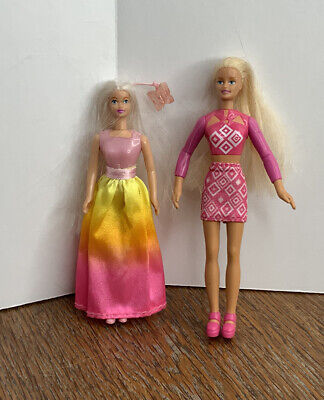A detailed image description captures two Barbie dolls standing on a brown and light gray wood-grain table, positioned against a folded white poster board serving as a background. The poster board has a visible vertical crease running from top to bottom.

The Barbie on the left features long blonde hair styled up and cascading down her back. She is dressed in a pink halter top with full sleeves, ending just below her breasts. Her outfit features a distinctive pink diamond pattern; the top displays an open circle in the middle of her chest, bordered by thick straps. Her midriff is visible beneath the top. She wears a short pink skirt, adorned with a similar diamond pattern, tapering into a pink Mary Jane-style shoes. This Barbie exudes an early 80s or vintage essence with her intricate attire.

The Barbie on the right is slightly shorter and possesses platinum blonde hair, parted in the middle and styled back. She wears a dress with a pink top and a vibrant gradient skirt that transitions from yellow at the waist to orange and then pink at the bottom. Her facial features include dark pink lipstick, blue eyes, and orangish eyebrows, with a gentle smile. A plastic butterfly accessory is attached near her head, adding a whimsical touch.

Both Barbies lean against the poster board background, which takes up most of the upper section of the image, highlighting the white surface with slight hints of an orangish-brown hue. The display, with its rough wood-grain table and neatly styled dolls, creates a nostalgic scene reminiscent of earlier decades, possibly from the 60s to early 80s.